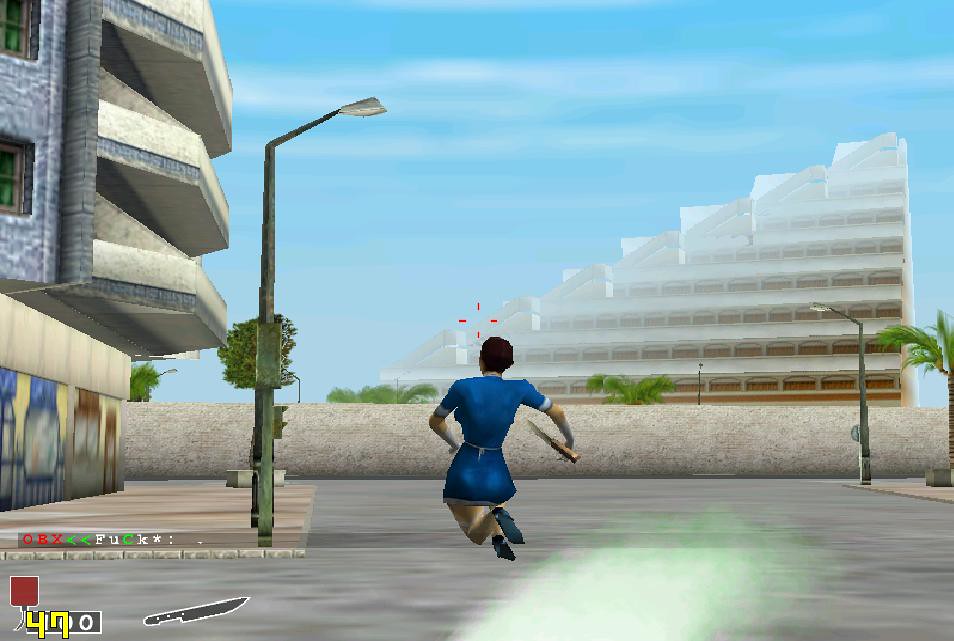This screenshot appears to be from a third-person action-adventure game, seemingly from the late 1990s to early 2000s, characterized by its low-resolution graphics and blocky polygons. It captures a woman in mid-air, likely caught in the midst of a jump. She is donning a retro nurse's outfit with a short skirt, reminiscent of styles from the 1940s and 1950s. Clutched in her right hand is a knife, adding a hint of danger to her appearance. A crosshair hovers just above her, indicating the player's aim. The setting appears to be an open city environment. On the bottom left corner of the screen, the user interface displays an image of a knife with the number 47 superimposed on it, possibly signifying the quantity of items or a score.